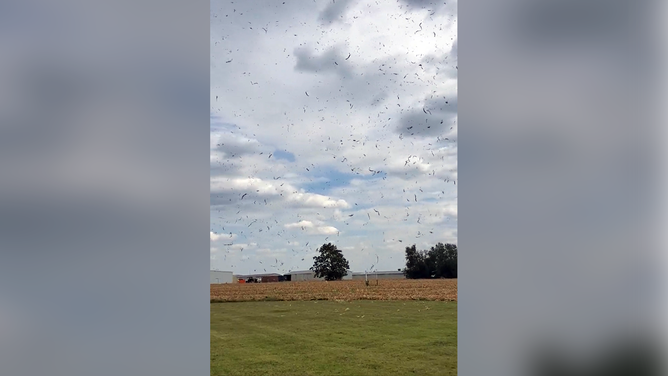This color photograph, presented in portrait orientation, captures a picturesque outdoor scene. The main image is displayed on a larger, blurry background of the same scene, giving the photograph a focused and framed look. At the forefront, lush green grass spreads out, leading to a section of the field filled with golden-hued harvested items, and beyond this, we see stacks of hay and various farm equipment. Birds are scattered across the sky, with some defined enough to discern their shapes against the backdrop of puffy white clouds and blue sky. The horizon is marked by a line of trees, including a prominent large tree on the right, another central tree, and a small white building to the left. The scene is grounded by a subtle hill or mountain range in the distance, contributing to a sense of depth and tranquility.